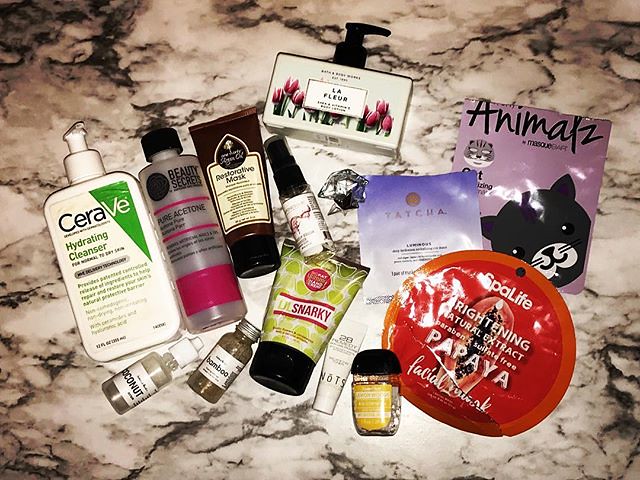The photograph showcases an eclectic assortment of 11 different cosmetic items arranged haphazardly across a marble table. Each product, ranging from hand pumps to disposable pouches and resealable tubes, is displayed flat on its back, with the tops tipped forward to reveal detailed labeling. Brand names like CeraVe are prominent, alongside mentions of ingredients such as papaya, and even imagery of animals. The cosmetics, all seemingly brand new, feature a variety of text and designs on their packaging. The image has a slightly washed-out appearance with dim lighting and a subtle muddiness effect around the edges, which contributes to the overall chaotic impression. The marble background blends with the products, making some items less distinct against the busy backdrop.